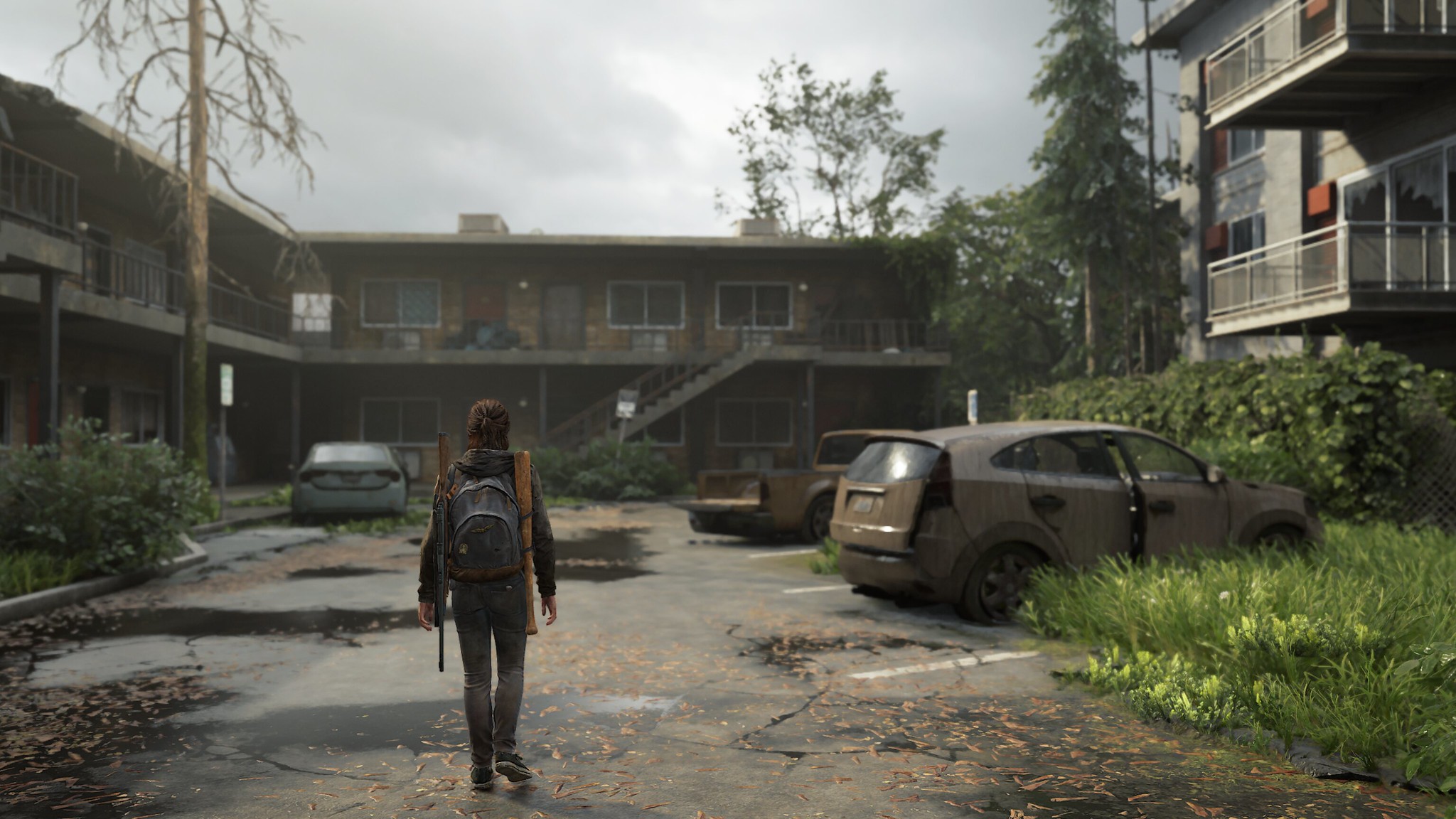The image is a screenshot from a video game, depicting a post-apocalyptic outdoor scene featuring a neglected two-story L-shaped motel on the left and a three-story apartment building on the right. The atmosphere is somber, characterized by an overcast gray sky hinting at a recent storm. The ground is littered with leaves, puddles, trash, and overgrown vegetation.

In the foreground, a female figure with short brown hair tied in a ponytail walks through the desolate parking lot. She is dressed in gray jeans, a gray long-sleeve sweatshirt, and carries a light blue backpack with brown accents, as well as a baseball bat and a gun with a light brown stock strapped to her back.

The parking lot is marred by cracks and dotted with abandoned, rusted vehicles, including a white car with its door ajar and a dark brown pickup truck with its tailgate open. Additional details include light green grass breaking through the concrete, dark green trees flanking the buildings, a blue and red curtain visible in the apartment windows, and gray and white railings on the balconies. The overall scene resonates with themes of abandonment and survival, emblematic of the setting in "The Last of Us."